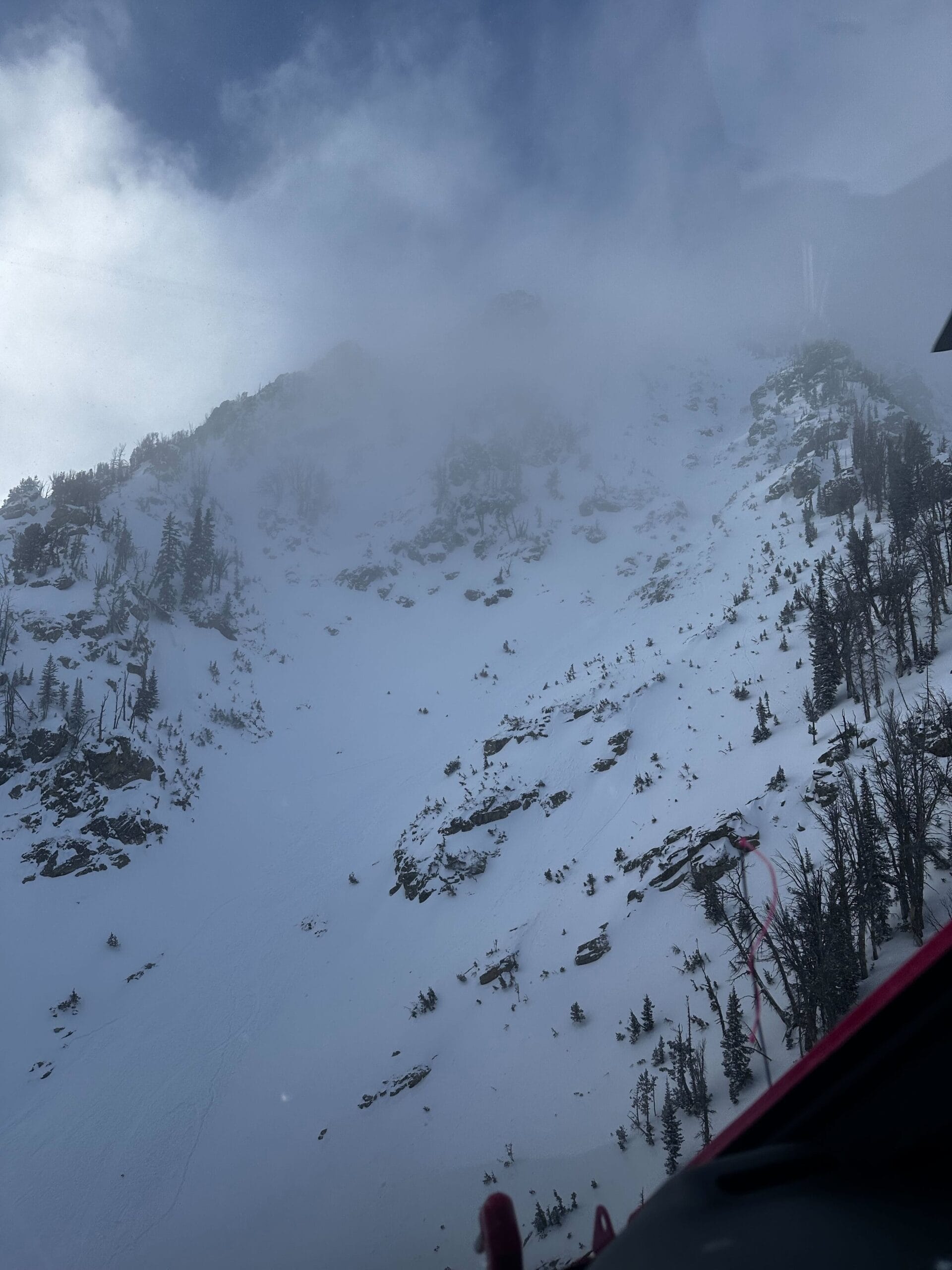This outdoor daytime photograph captures a striking view of a snow-covered mountain slope. The rectangular image, measuring approximately five inches in height and four inches in width, showcases a steep incline that dominates the frame. Sparse pine trees dot the left and right sides of the mountain, while the center features a smooth expanse of flat snow leading towards the lower left corner. A curious detail is found in the lower right-hand corner: a black canvas material with a pink edge, positioned about an inch from both the bottom and right edges.

The top of the mountain is shrouded in clouds, obscuring the peaks and blending them with the dark gray sky or mist above. This composition suggests that the photo may have been taken from a vantage point high up, possibly from a ski lift or gondola. The interplay between the smooth snowy center and the rocky, tree-speckled sides of the mountain, alongside the enveloping clouds, creates a dramatic and immersive alpine scene.